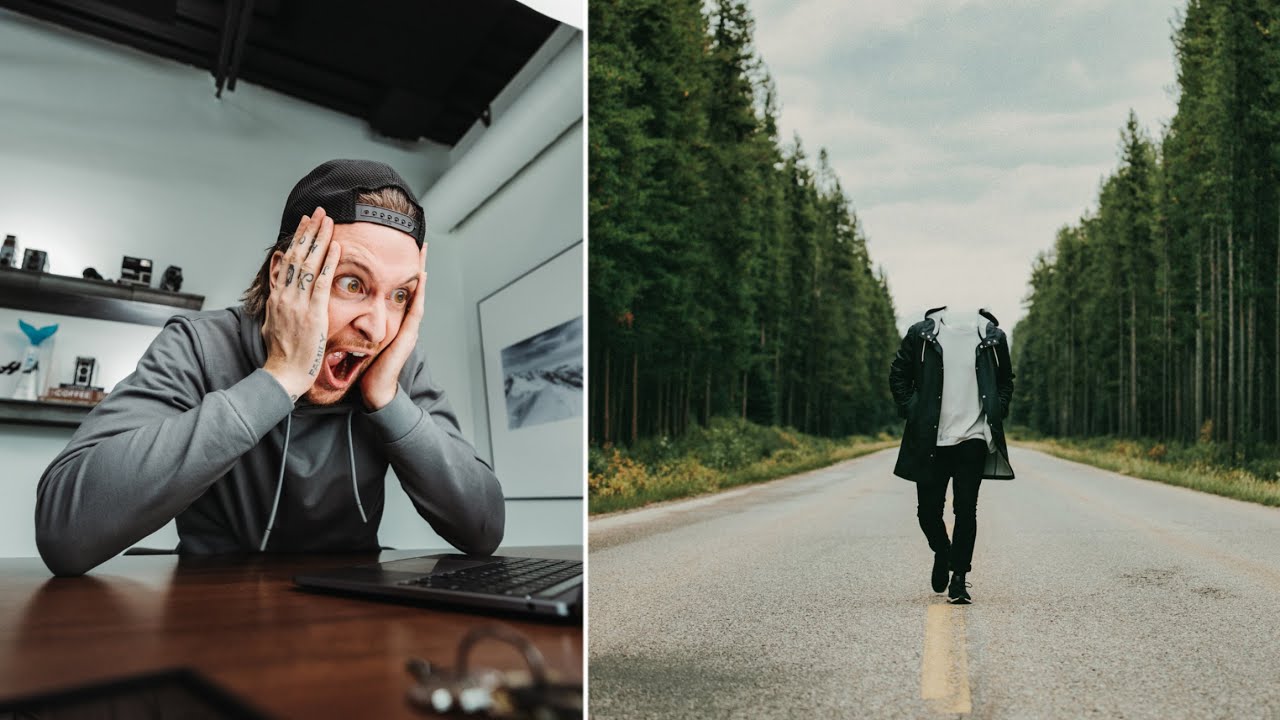This side-by-side image comprises two distinct photographs. On the left, there is a man seated at a wooden table in a white room with black floating shelves and a black-accented ceiling. He is in front of a laptop, both hands pressed against his cheeks, exhibiting an exaggeratedly shocked expression with his wide eyes and gaping mouth. Dressed in a gray sweatshirt and a black baseball cap worn backwards, he appears utterly stunned by what he's viewing on the screen. The right-hand photograph features a headless figure clad in a long green jacket, white sweatshirt, black pants, and black shoes, walking down the center of a tree-lined road. The absence of the man's head and the context given by the left image suggests that the man is reacting to the mysterious, headless figure on his laptop.